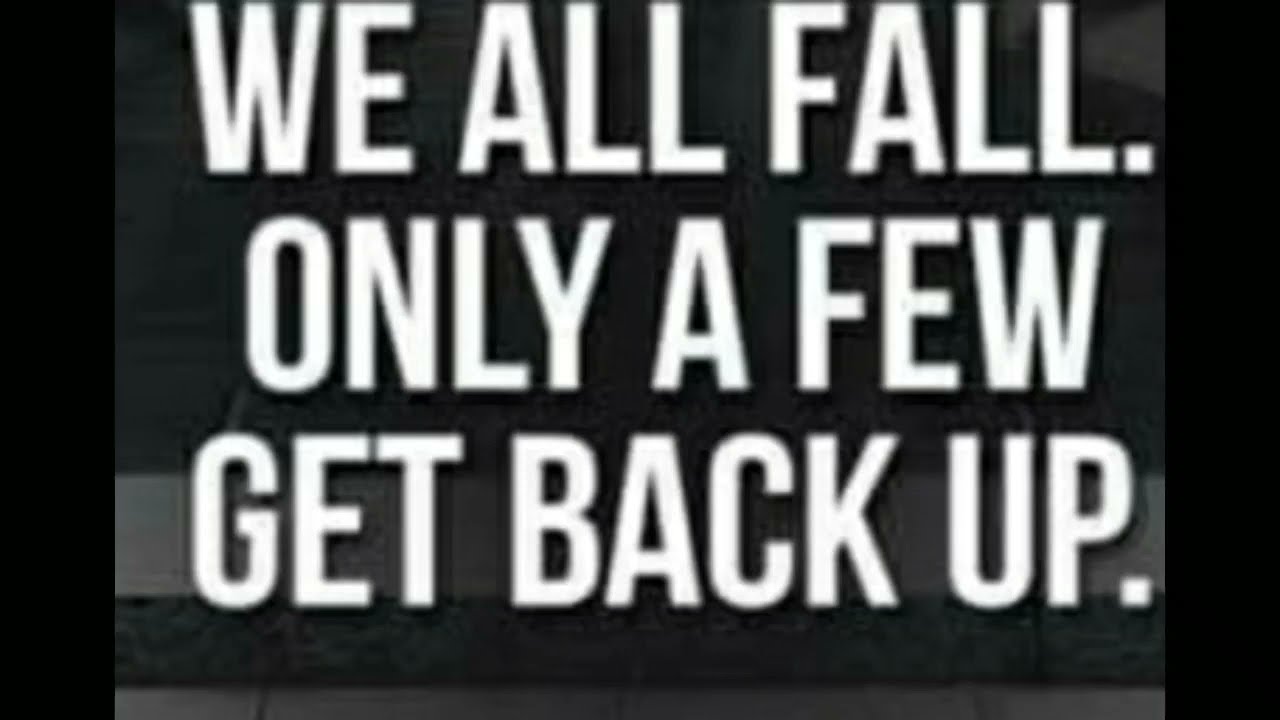The image presents a pixelated, black-and-white graphic with a motivational statement in large, capitalized, white block letters. The text spans three lines: "WE ALL FALL." on the first line, "ONLY A FEW" on the second, and "GET BACK UP." on the third, each phrase punctuated with a white square period. The background reveals a blurred, grayscale scene featuring a sidewalk flanked by patches of grass. The top portion of the image is darker, transitioning to a lighter hue at the bottom. The image is bordered on the left and right by thick, vertical black strips, adding to the overall monochromatic aesthetic.